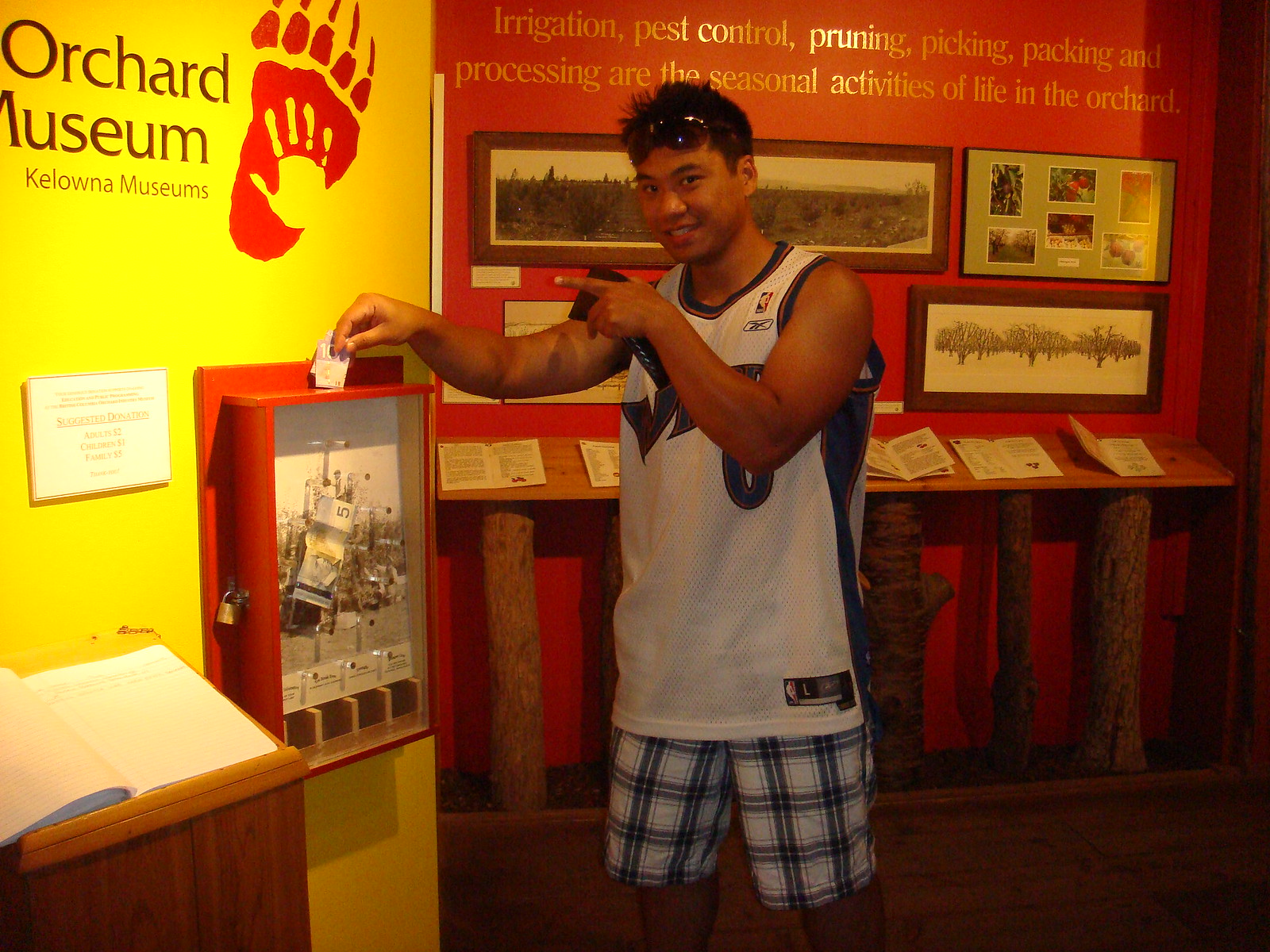In the photo, a man dressed in a basketball jersey and shorts can be seen inserting a piece of currency into a transparent donation box. The box reveals various other donations inside, suggesting a collective effort for a cause. Behind him, the wall displays the text "Orchard Museum, Kelowna Museums," indicating that the location is a museum dedicated to orchard life. To the right of the man, there is an educational exhibit that highlights different types of trees. At the top of this exhibit, there is informative text listing the seasonal activities associated with orchard life: Irrigation, Pest Control, Pruning, Picking, Packing, and Processing. The scene captures a moment of philanthropy amidst the rich, educational backdrop of the Orchard Museum.